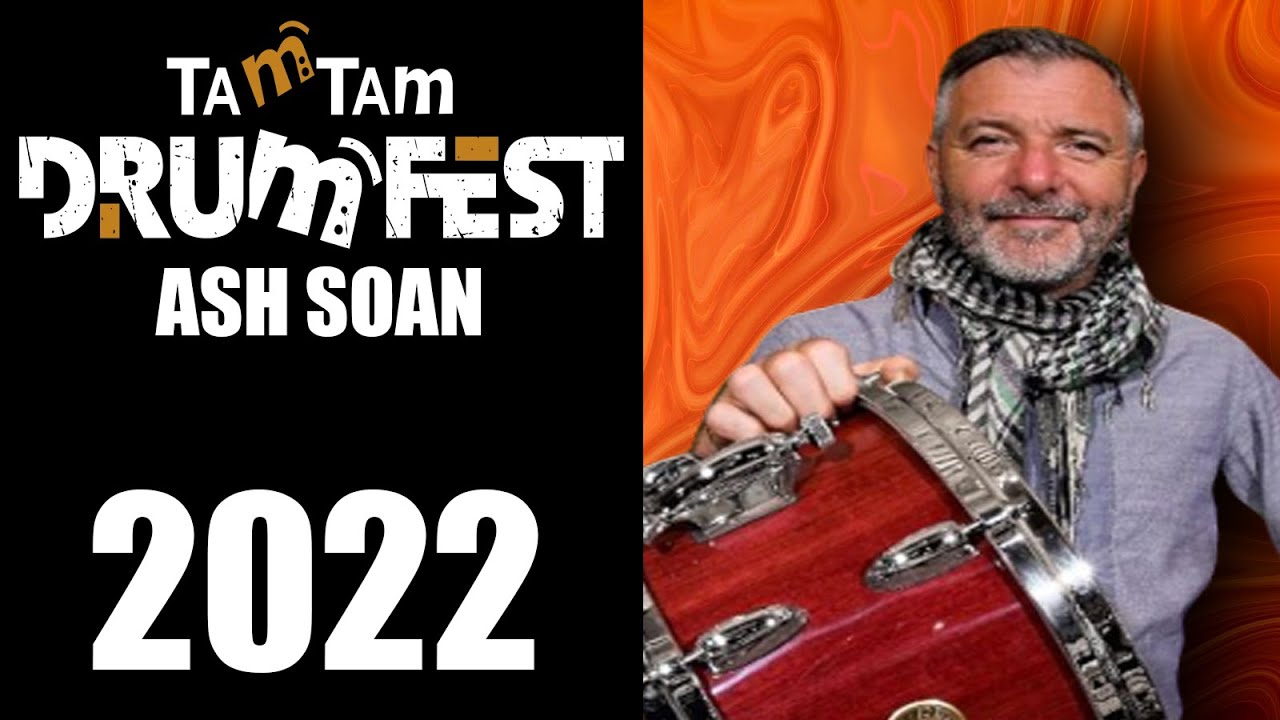The image is a rectangular poster that looks like concert signage. The left side of the poster has a black background featuring the text "Tam Tam Drum Fest Ash Soin 2022" in a white font with brown accents, especially the "M" in "Tam" which is angled and in brown. The right side shows a photograph of Ash Soin, a man possibly in his 50s or early 60s with a ruddy complexion and salt-and-pepper hair and goatee. He is wearing a long-sleeved gray sweater and a black-and-white checkered scarf around his neck. Ash Soin is smiling at the camera with his hand resting on a drum that has a cherry reddish-brown body and silver trim. The background behind him features an orange, swirly, psychedelic pattern that resembles molten lava or liquid. All colors and text have been noted in detail.